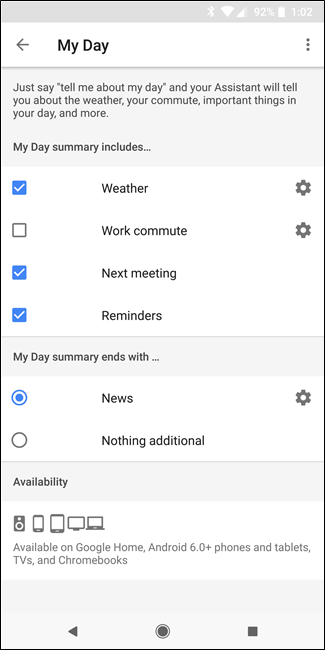This is a somewhat blurry screenshot of a phone screen featuring a voice assistant settings page. Despite the blur, you can identify it as a phone screen due to the typical phone information displayed at the top right corner, which includes the time "1:02" and a battery icon showing a 92% charge.

The top of the screen prominently features the title "My Day." Below this, there's a prompt that reads, "Just say 'Tell me about my day,' and your Assistant will tell you about the weather, your commute, important things in your day, and more." This indicates that the screenshot is indeed from a voice assistant settings page.

Further down, a section titled "My Day Summary includes" lists several elements with checkboxes next to them. The listed items are:
1. Weather (checked)
2. Work Commute (unchecked)
3. Next Meeting (checked)
4. Reminders (checked)

Following this, there's a section labeled "My Day Summary ends with," offering two options:
1. News (selected)
2. Nothing additional

So, the chosen configuration ends the daily summary with news updates.

At the bottom of the screen, the "Availability" section shows various device logos, indicating that the assistant is available on Google Home, Android 6.0+ phones and tablets, TVs, and Chromebooks.

Finally, the navigation bar at the bottom of the screen displays the back button, home button, and all apps button, confirming the interface is that of a smartphone.